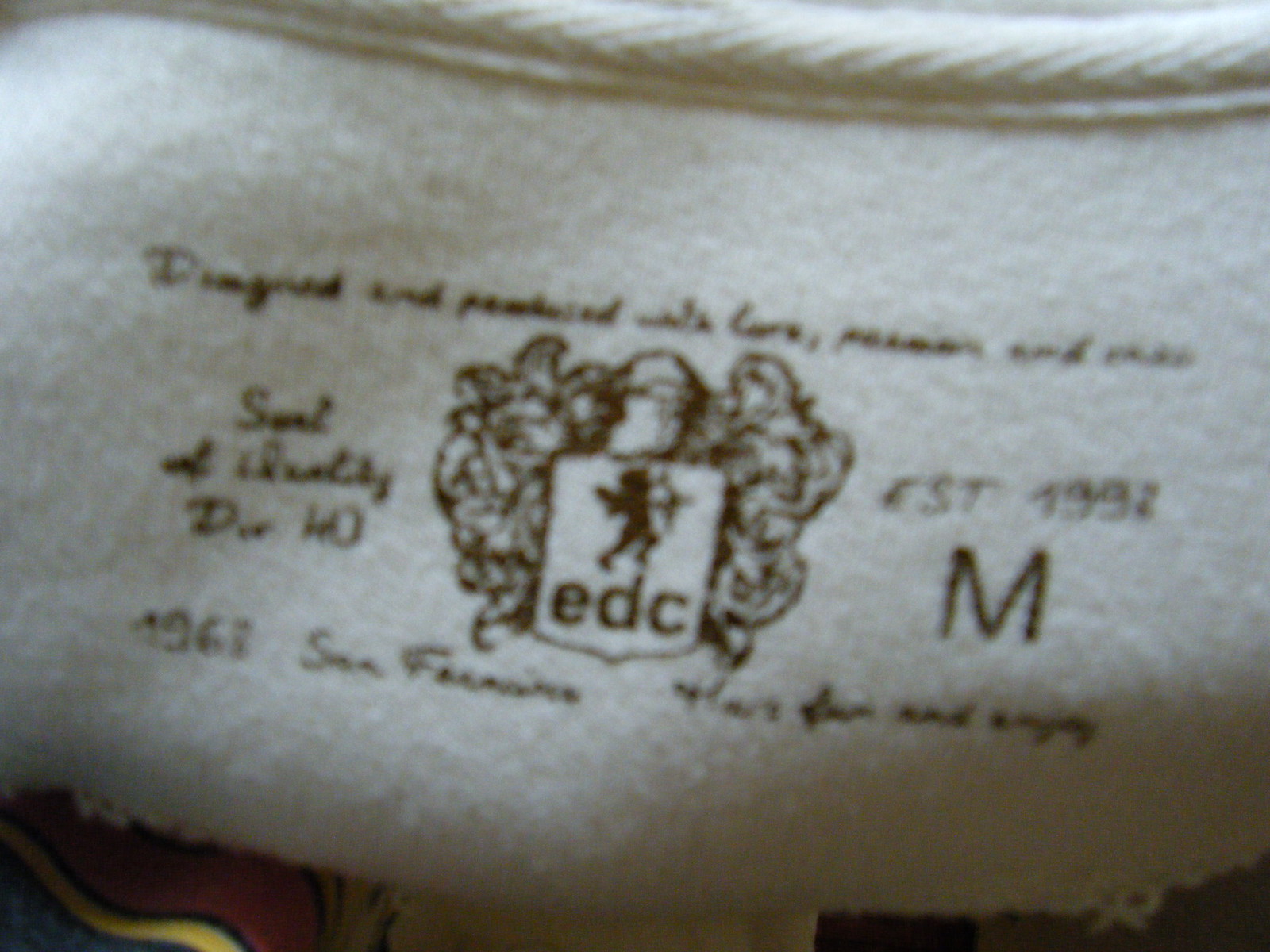This image is a landscape-oriented close-up shot that is somewhat out of focus, rendering the finer details indistinct. The primary subject appears to be a piece of white fabric, identifiable by its texture. At the top of the image, there is a hemmed edge of the fabric, further emphasizing the fabric's texture. Despite the blurriness, black printed details are visible on the fabric, suggesting that it is likely an internal label from a piece of clothing. Prominently displayed in the center is a seal featuring the icon of a cupid inside a shield, accompanied by the letters "EDC." To the right of this seal, a large "M" can be discerned, indicating that the garment is probably size medium.